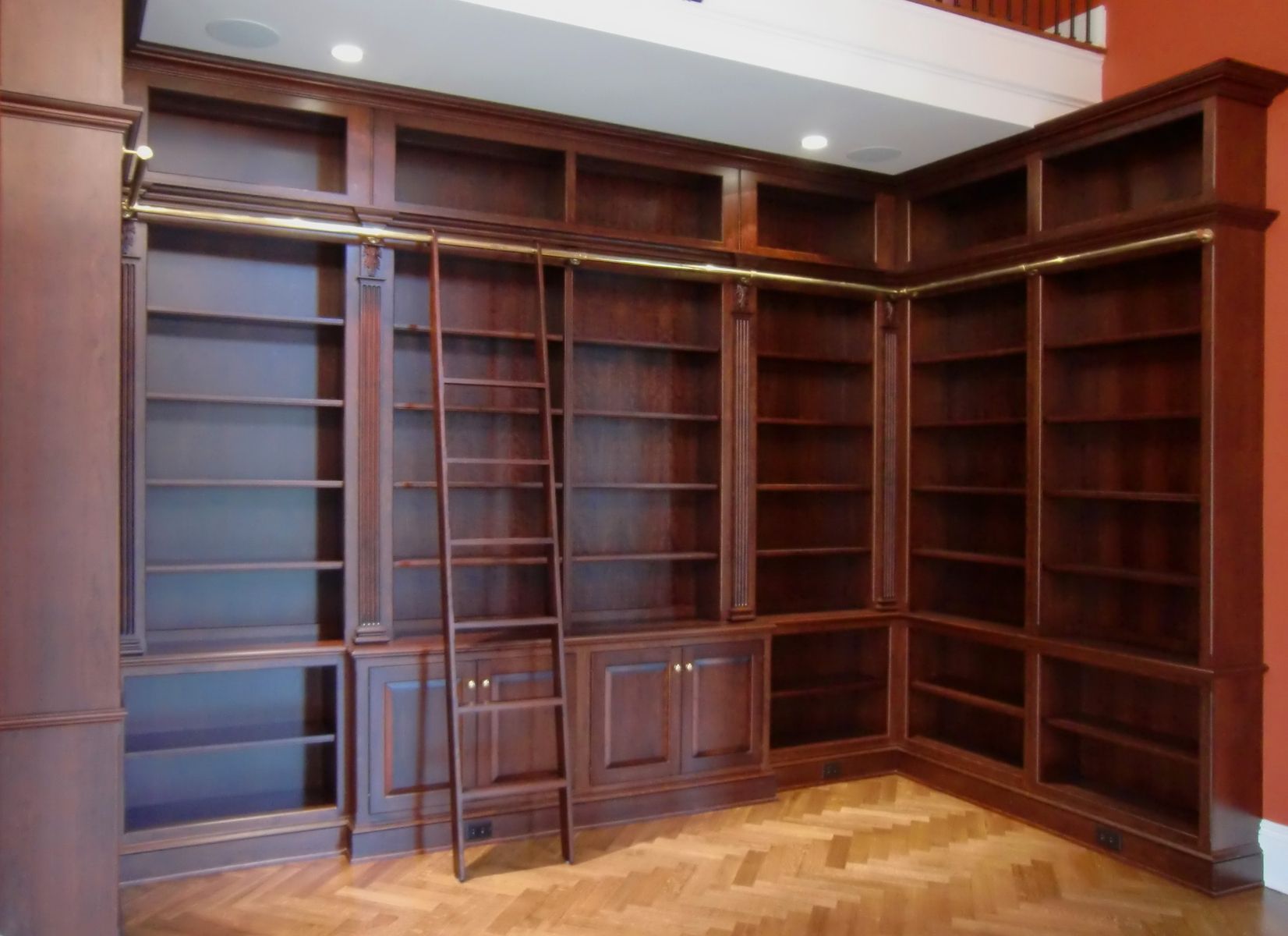The image depicts an empty personal library or den with built-in, dark cherry brown bookshelves arranged against three walls in a U-shape. The shelves extend from floor to ceiling, with a golden rod running across the top to support a ladder which allows access to higher shelves. The ladder stands in front of one of two small cabinets situated at the bottom of the central bookcase on the far wall. The backdrop wall is a reddish-orange hue with visible white baseboards, and the floor features a tan and brown herringbone pattern. Overhead, a white ceiling houses two recessed lights and two circular vents. Above the shelves, there is an elevated platform, and a railing suggests the presence of a second-floor overlook.